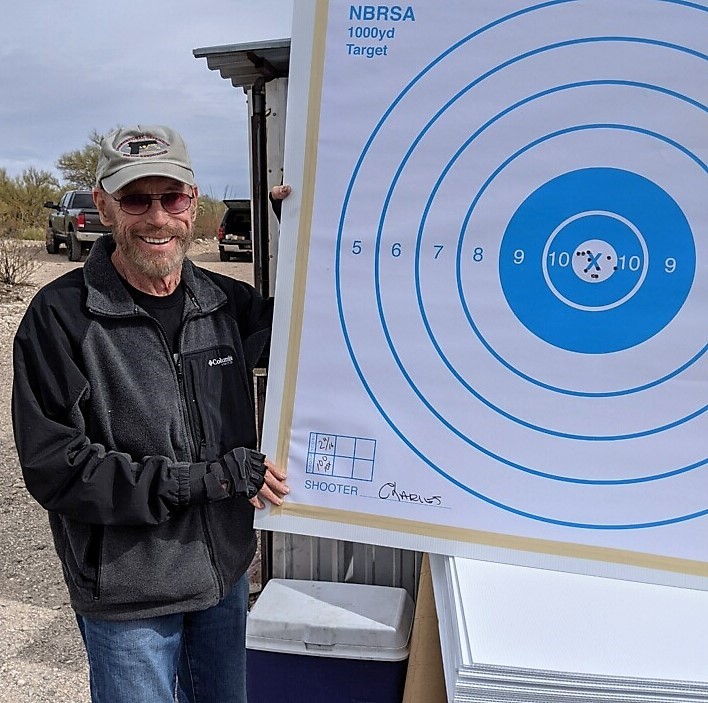This photograph features a white male, possibly in his early 50s, standing outdoors in a woodsy or country setting. He is wearing a gray baseball cap, sunglasses, and a black t-shirt underneath a black and gray zip-up fleece jacket. He sports a thick beard and mustache and is dressed in light blue jeans. The man is holding a large rectangular sign with a white and blue bullseye target printed on it. In the upper left-hand corner of the sign, it reads "NBRSA, 1,000-yard target" in blue. The background includes a couple of vehicles—one being a pickup truck—parked near a blue and white cooler, along with a backdrop of trees and a gray, slightly cloudy sky. The man appears to be smiling as he presents the target.